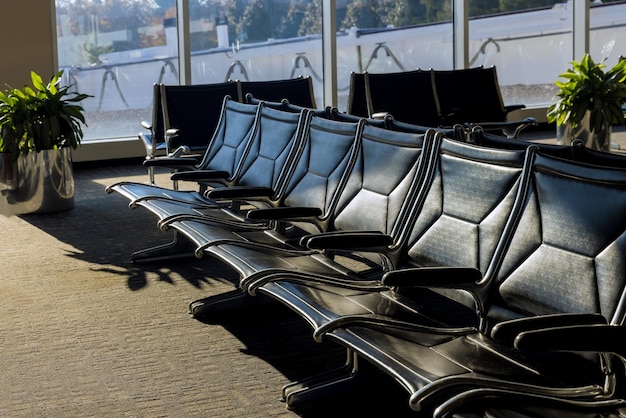The image depicts a waiting area, likely an airport, featuring a row of six black seats made of vinyl or leather-like material, each separated by thin armrests. This row is arranged back-to-back with another set of identical seats, creating doubled layers of seating. The hexagonal pattern on the backs of the chairs adds a subtle design touch. The floor is covered in a gray carpet, which extends throughout the room. In the back left and back right corners, large silver planters house vibrant green plants. The background features five tall, wide windows offering a view of a divider wall and some trees outside, emphasizing the interior setting.